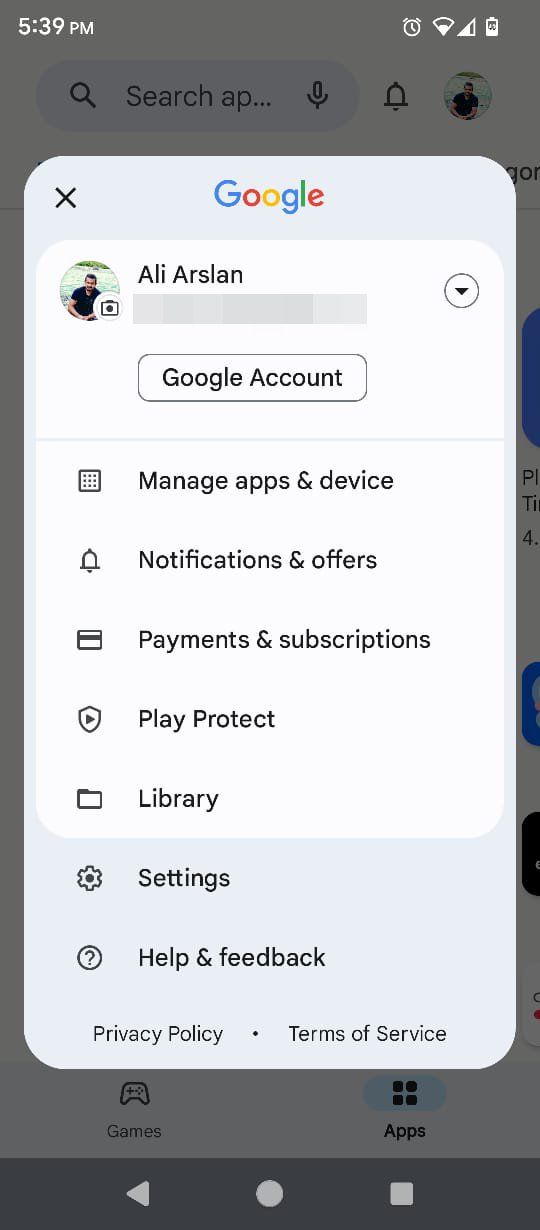### Detailed Captured Image Description:

The image is a screenshot of a mobile device displaying an overlay window for managing a Google account. The overlay window occupies a significant portion of the screen vertically, with a large rectangular area. In the top-left corner of the overlay, there is a small "X" button which allows the user to close the window.

At the top of the overlay, the word "Google" is prominently displayed. Below that, the user's profile picture and name are shown, although some of the information beneath these elements is obscured by gray squares, likely for privacy reasons.

Immediately below the blocked-out information, there is a "Google Account" button. Following this button, the overlay contains various sections denoted by small icons. These sections include:

- **Manage Apps and Devices**
- **Notifications and Offers**
- **Payments and Subscriptions**
- **Play Protect**
- **Library**
- **Settings**
- **Help and Feedback**

At the very bottom of the overlay, there are additional links for accessing the **Privacy Policy** and **Terms of Service**. 

All these features are laid out in a user-friendly manner, allowing easy navigation and management of the Google account.